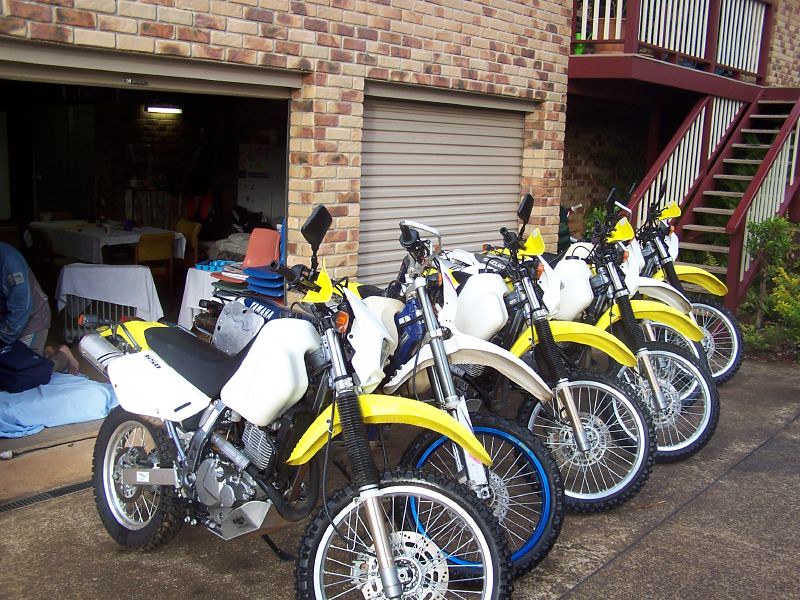The image captures an outdoor scene in front of a brick, two-door garage. The left garage door is open, revealing the interior cluttered with items such as plastic chairs, while the right garage door remains closed. In front of the open garage door, six motorcycles are lined up side by side, all positioned in a profile view with their wheels angled from the upper left to the bottom right of the image. The first and third motorcycles feature a striking white color with yellow fenders, while the second motorcycle differs with its entirely white exterior and white fender. All motorcycles are equipped with black seats. Additionally, the side view of a man kneeling on a mattress covered in blue linen can be seen near the open garage door. To the side of the garage, a staircase ascends, presumably leading up to the building above.